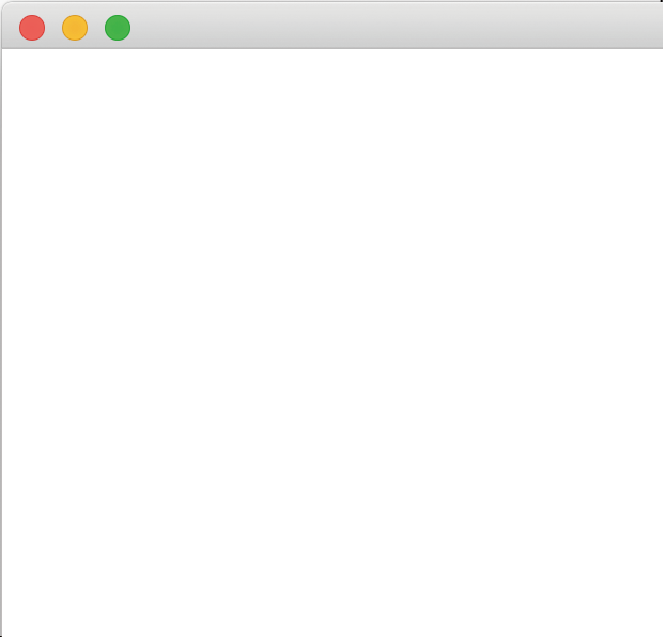In the image, a minimalist screenshot is displayed in the upper left corner against a gray banner. Centered within the banner are three equally-sized circles, each representing primary colors in the following order from left to right: red, yellow, and green. The rest of the header above these circles is a light gray hue. Below the banner, the screen transitions to a pristine white with a narrow gray border running vertically along the left side and continuing along the top. Additionally, a horizontal gray line matching the banner's shade is positioned immediately beneath the circles. Consequently, the image features a total of three distinctive light gray lines framing the elements.